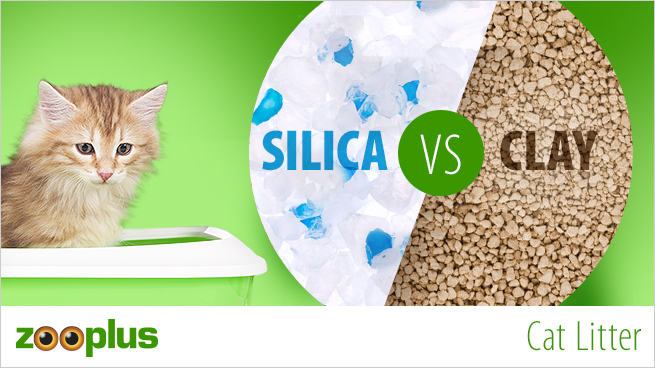This advertisement for Zoo Plus Cat Litter features a detailed comparison between silica and clay cat litter types. The background is a vibrant grassy green, seamlessly extending into the green litter box where a small tabby cat sits, looking downward. The bottom left corner prominently displays the Zoo Plus logo, with the O's cleverly designed as eyeballs, just above the label "cat litter" contained within a white-bordered strip. On the right side of the image, a circular comparison highlights two types of litter; white and blue synthetic materials are labeled 'silica,' while tiny beige pebbles represent 'clay.' The words "silica versus clay" emphasize this juxtaposition, allowing viewers to easily compare the different cat litter options.